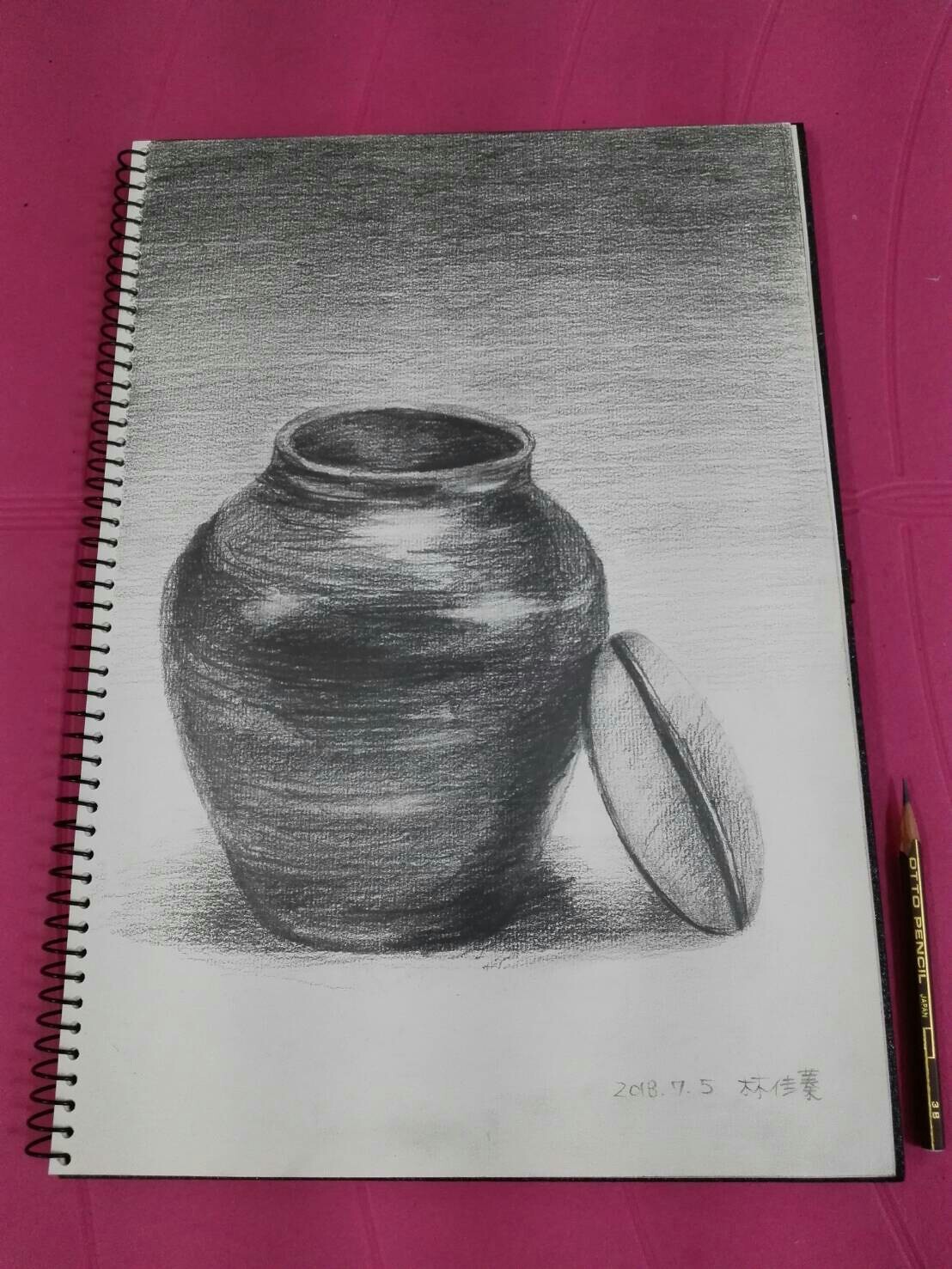Overhead view of a bright purple table surface featuring a short black pencil with tiny, unreadable white text on its side, placed in the corner. Dominating the scene is a spiral-bound sketchbook opened to a page displaying a meticulously detailed pencil sketch. The sketch depicts a vase or urn with the lid removed and leaning against its side, rendered with intricate shading and highlights.